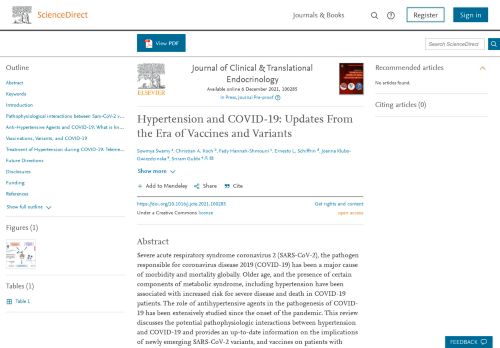Here is a revised and detailed caption for the image described:

"A screenshot from the ScienceDirect website, showing a clean and organized layout primarily in a three-column format. At the top bar, options such as 'See journals and books,' 'Register,' and 'Sign up' are visible. On the left side, there is an outlined section with numerous links displayed in blue text, possibly labeled as 'Abstract' and 'Keywords.' Due to the small and blurry nature of the text, further details are obscured. Near the bottom, a small graphic can be seen, but its contents are unclear. Below the top bar, a blue button labeled 'View PDF' is present, accompanied by a PDF icon on its left. To the right of this button, there's a search option. Towards the center, partially legible text seems to reference the 'Journal of Clinical Translation Endocrinology,' featuring an image of a tree on what appears to be a book cover. The header reads, 'Hypertension and COVID-19: Updates from the Era of Vaccines and Variants,' followed by more blue option texts below. At the bottom center, there is an abstract section, though details are indistinct. To the far right, another recommended book is displayed. The screenshot’s overall presentation appears to be text-heavy, with clear and organized content distribution, sadly marred by the small and blurry text which hinders readability."